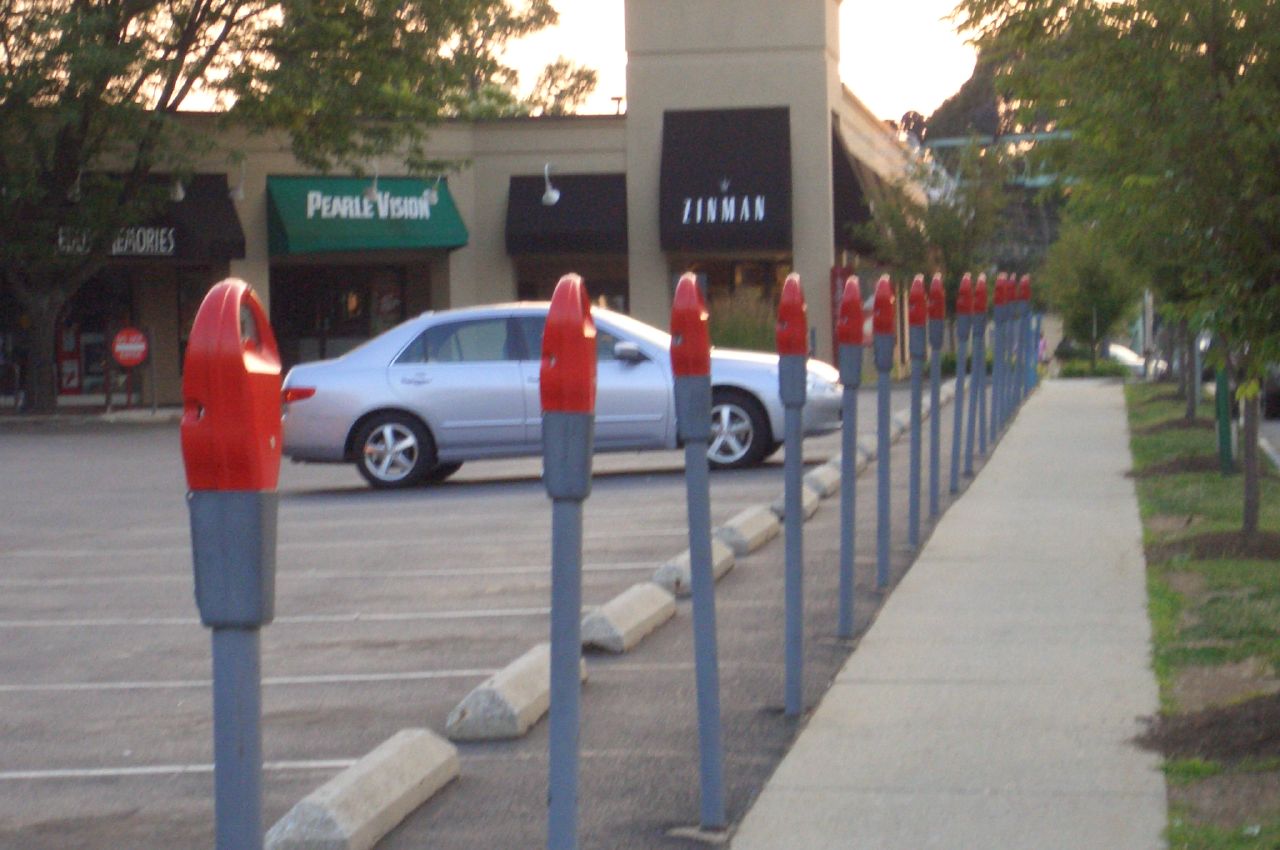The photo captures the serene atmosphere of a parking lot adjacent to a shopping center or mall during either sunrise or sunset. Central to the background is a Pearl Vision store, flanked by a store named Zenmon on one side. Another storefront, partially obscured by a tree, has the visible word "Memories." The parking lot features a silver sedan parked alone in an otherwise empty row of spaces, each equipped with parking meters characterized by gray poles, gray bottoms, and red tops. Behind the parking meters runs a sidewalk, bordered by a grassy area with several trees lining its perimeter. In the far background, a person wearing a pink shirt is walking, adding a touch of human presence to the tranquil scene.